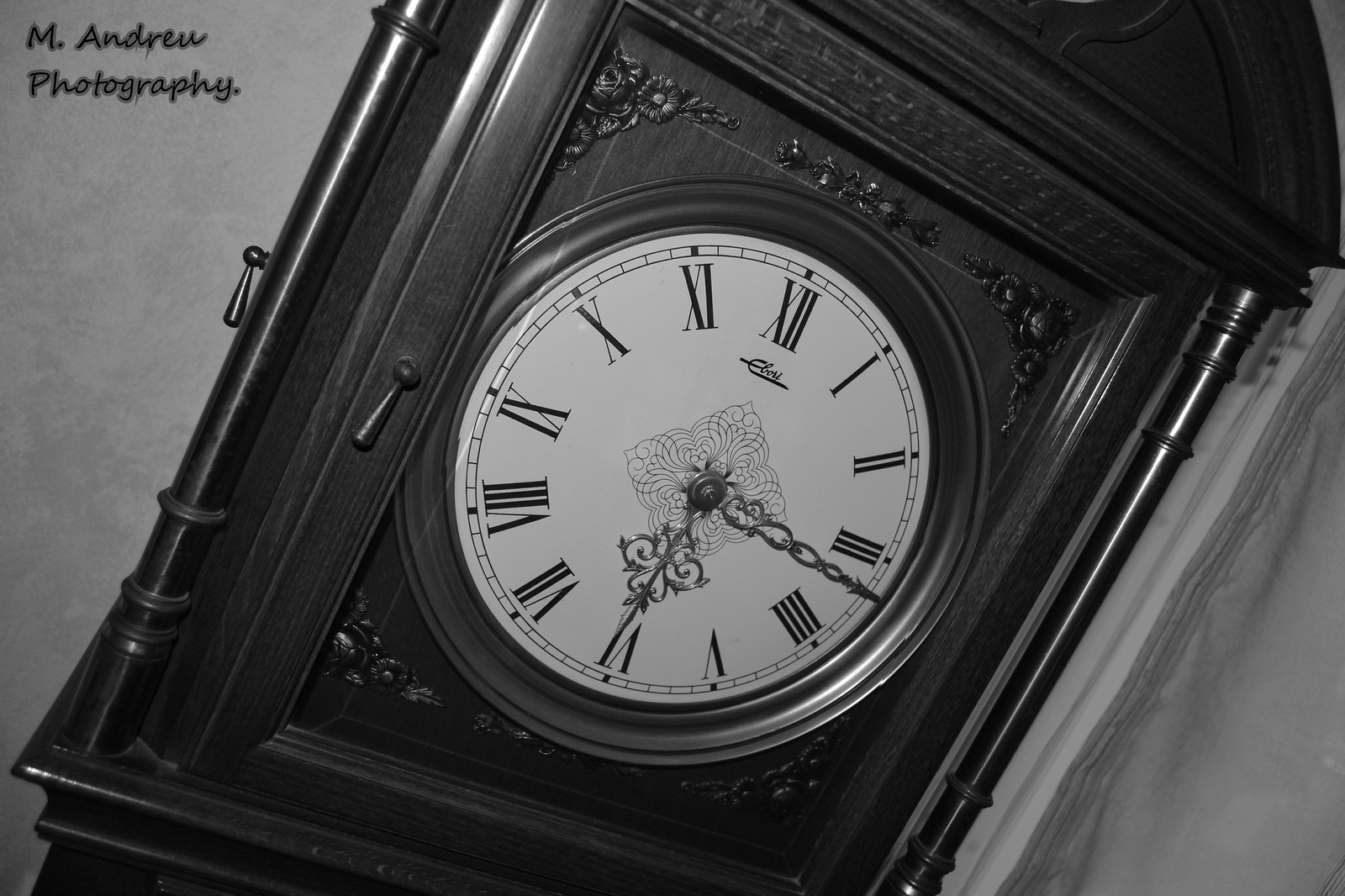This captivating black and white photograph, taken by M. Andrew Photography as indicated in the upper left corner, showcases the ornate top section of a monumental grandfather clock. The backdrop is a gray wall, emphasizing the classic and timeless feel of the image. To the right of the clock, a drapery or similar material subtly enters the frame, adding a soft texture contrast. 

The most striking feature of the clock is its large, intricately designed face. The face boasts a white background with a scalloped, diamond-shaped motif at its center, from which several concentric circle patterns emanate. The clock hand indicates the time as approximately 6:17, and both hands are adorned with delicate, scalloped designs, including a diamond embellishment on the smaller hand.

Encircling the clock face are beautifully carved wooden details, adding to the grandeur and aged elegance of the piece. Roman numerals are used to mark the hours, providing a classic touch. Beneath the 12 o'clock position, a small, intricately inscribed company name can be faintly seen. Completing its functional and aesthetic design, the clock features dual pulls — one prominently visible and another situated behind it — for accessing the clock's inner workings.

The photograph, taken at an angle, emphasizes the depth and dimensionality of the clock, highlighting its historical and artistic significance.